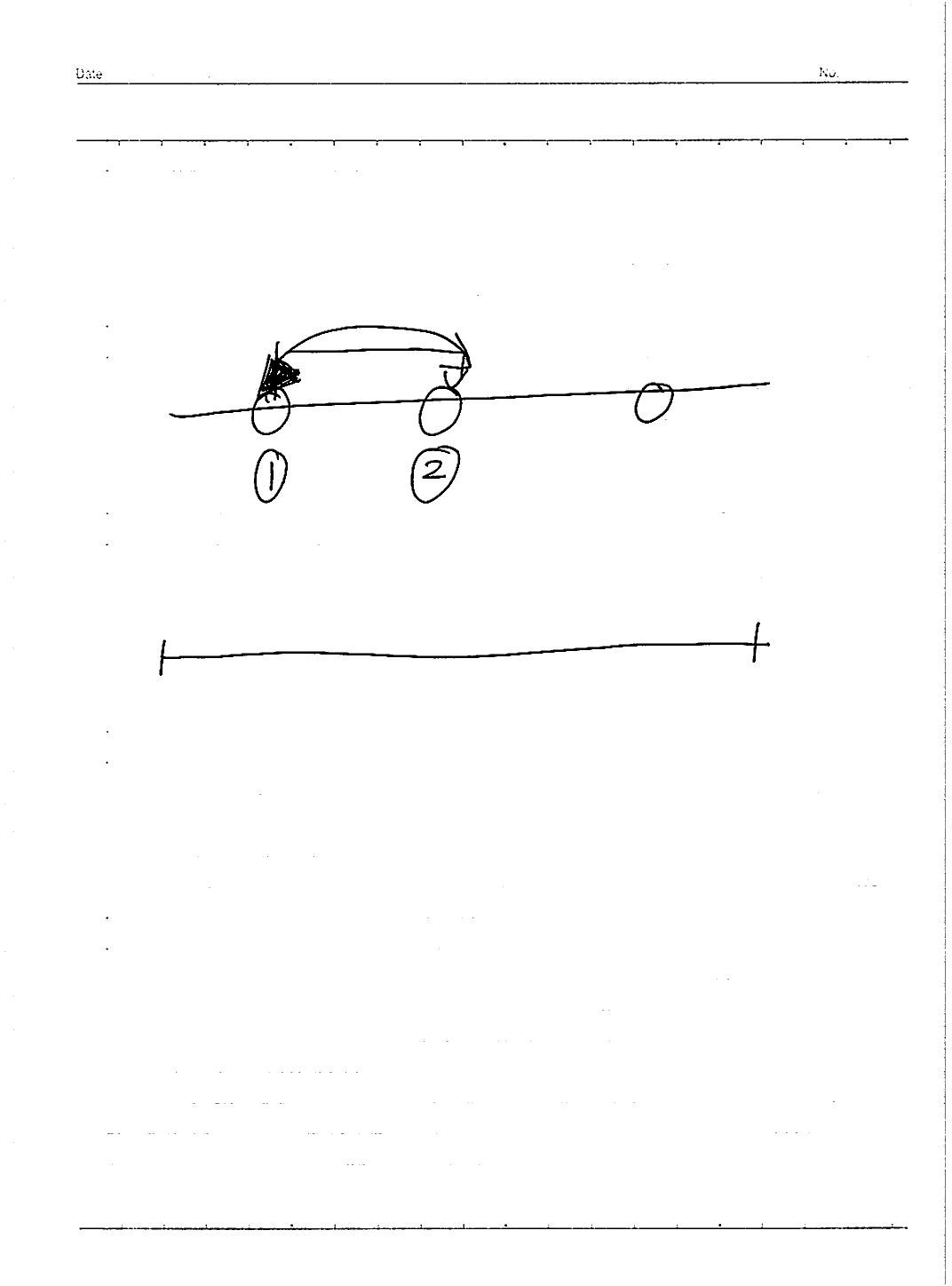The image displays a white piece of paper featuring various printed and hand-drawn elements. At the top of the paper, there's a printed scale resembling a ruler. Above this black scale line, there's a blue line with barely legible text—likely indicating a space for the date and number, discernible by what appears to be "Date" and an "O" for number. 

At the bottom, another blue line is marked evenly like a hand-drawn ruler. Below this is a horizontal black line with three circles above it. Each circle houses the numbers "1" and "2," except the third circle, which is blank. Curved lines with arrows connect these circles; one has a solid black arrowhead, while the other has a curved hollow arrowhead. 

Beneath this arrangement, there's another line, resembling a scale, featuring a mark on the far left and another mark near the right end.